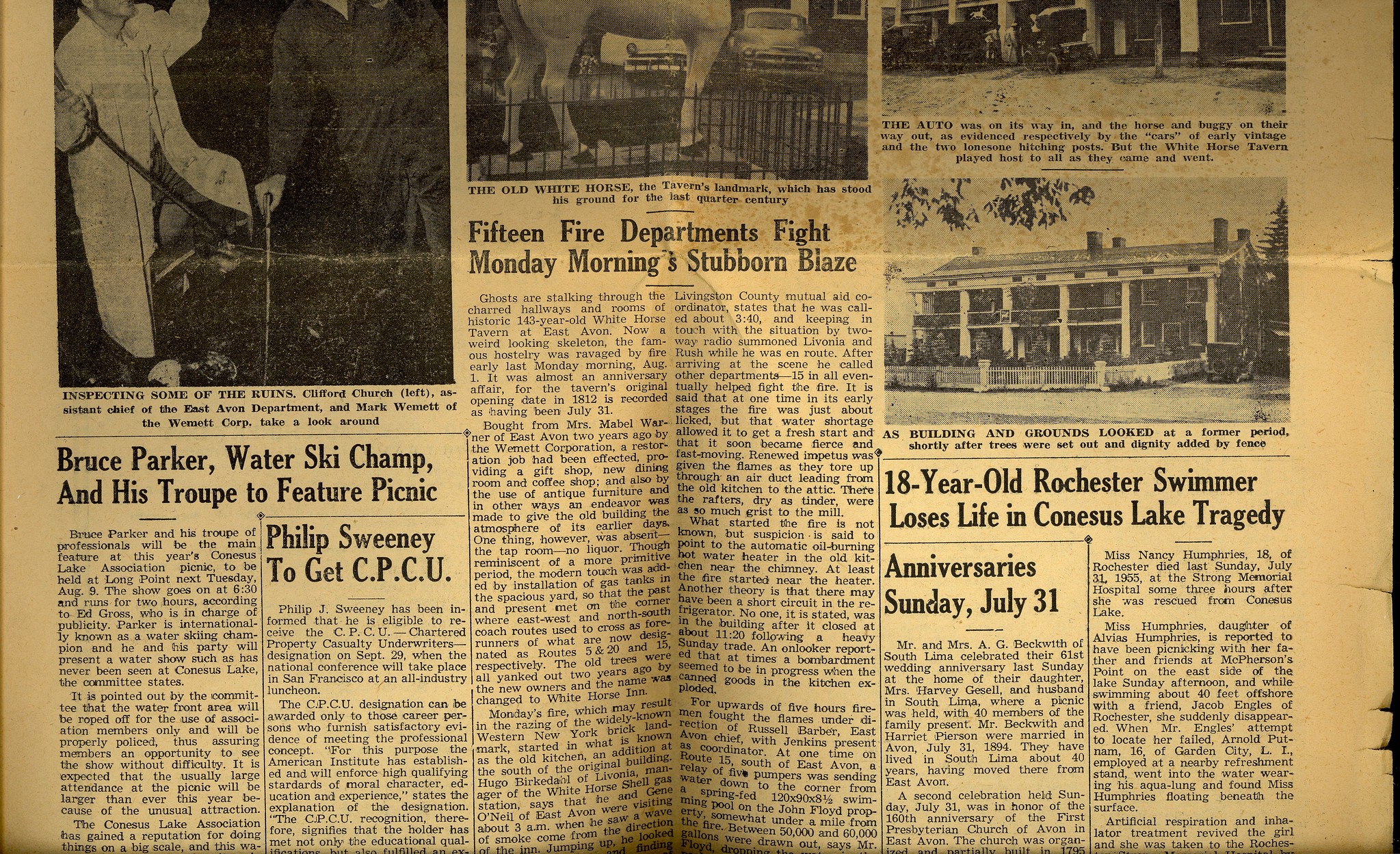This image shows a heavily worn and yellowed photocopy of an old newspaper, folded multiple times with evident creases. The newspaper is divided into three vertical columns with black-and-white photos at the top of each column. The left column headlines include "Bruce Parker, water ski champ, and his troop to feature picnic" and "Philip Sweeney to get CPCU." In the center column, a prominent headline reads "15 fire departments fight Monday morning stubborn blaze," with an image below captioned, "the old white horse the taverns landmark which stood his ground for the first quarter century." The right column features a headline stating "18 year old Rochester swimmer loses life in Conesus Lake tragedy" and mentions "Anniversaries Sunday July 31st." The newspaper's torn edges and overall oxidized, beige tone emphasize its age and fragility.